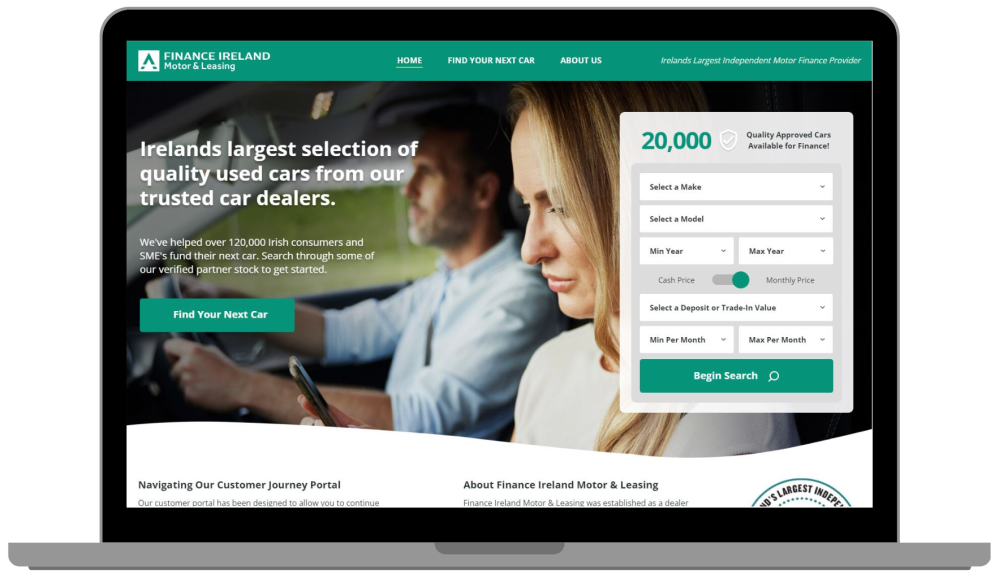Screenshot of a computer screen displaying a website dedicated to car financing and leasing in Ireland. At the top of the page, headings read "Finance" and "Ireland," followed by "Motor and Leasing." Below these headings is an image depicting a man driving a vehicle from the right-hand side, indicating a right-hand drive car. The man, who has a salt-and-pepper beard and darker hair, is dressed in a blue button-down shirt with sleeves rolled up. Beside him sits a middle-aged woman with brown hair and blonde highlights, attentively looking at her cell phone.

Overlaying the image is a bold white text proclaiming, "Ireland's largest selection of quality used cars from our trusted car dealers." Below the image, additional text states, "We've helped over 120,000 Irish consumers and SMEs fund their next car," and encourages visitors to "search through some of our verified partner stock to get started." At the bottom of the page, a prominent green button with white text invites users to "Find your next car."